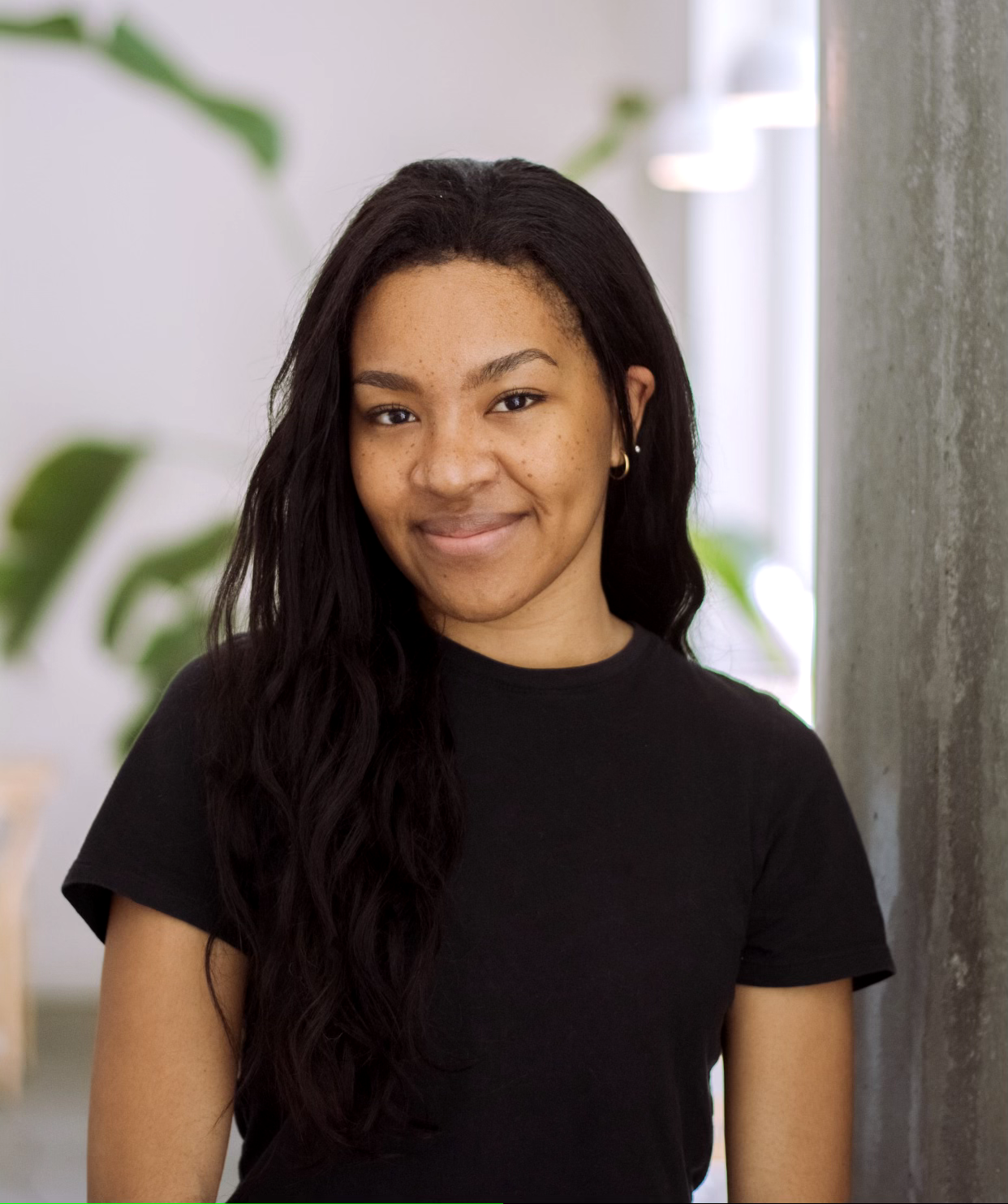In the image, a black woman with long black hair is wearing a black t-shirt and a small gold hoop earring in her right ear. She stands against a background that features a light purple wall decorated with green leaves at the edges. The right side of the frame shows a gray wall, while to her immediate left, slightly behind her shoulder, there is a window with a white frame, through which bright light streams into the room. This light accentuates the white window frame at the bottom near her shoulder and above her head. To the far left sits a brown chair. The room has gray flooring, adding a neutral base to the colorful yet serene setting.